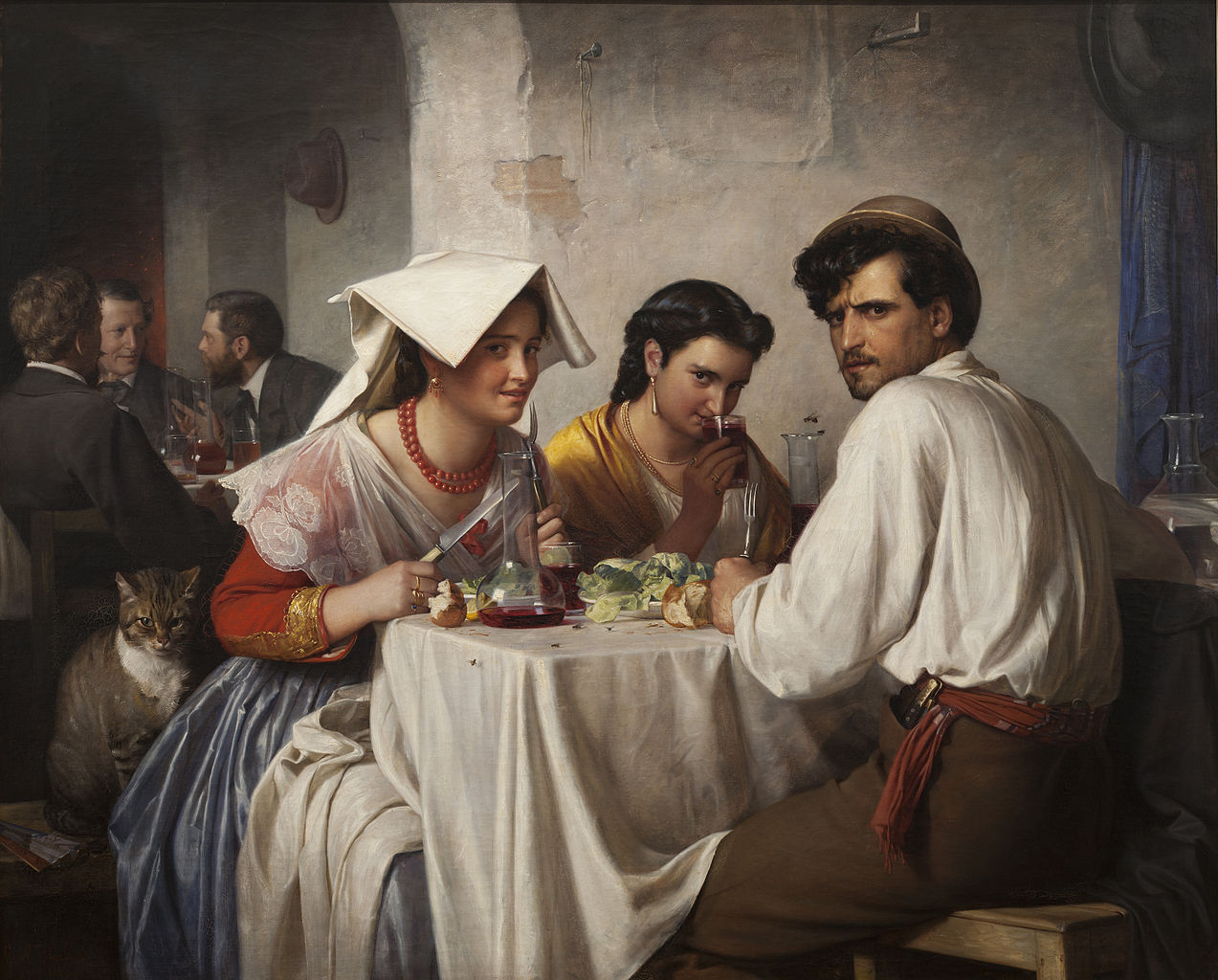This detailed painting features a small, intimate dining scene from what appears to be the 16th or 17th century, inferred from the characters' attire. In the foreground, three individuals are seated at a white table adorned with a realistic tablecloth. The central figure is a man in a white shirt, brown pants, and a cap, who gazes directly at the viewer with a somber expression. On his left, a brunette woman with a white angular headpiece reminiscent of a tent, wears a sheer scarf, a red dress, and a blue skirt. She holds a knife and fork in her hands. Adjacent to her, another brunette woman with black hair dons a gold shawl and is depicted sniffing a glass of red wine. This woman also wears earrings, lending a touch of elegance to her appearance. A brown and white tabby cat is perched nearby, providing a cozy domestic element to the scene.

Behind the trio, three men, all clad in business suits, are engrossed in conversation at another table. The backdrop features a gray, stone wall with white highlights, against which various objects like a hat and a clear bottle filled with red liquid are displayed. The painting's dramatic, realistic lighting enhances the detailing—especially notable in the intricate textures of the clothing, such as the man's shirt with its lifelike wrinkles and shadows. The overall composition exudes a blend of realism and historical ambiance, capturing a moment of shared human experience and interaction.